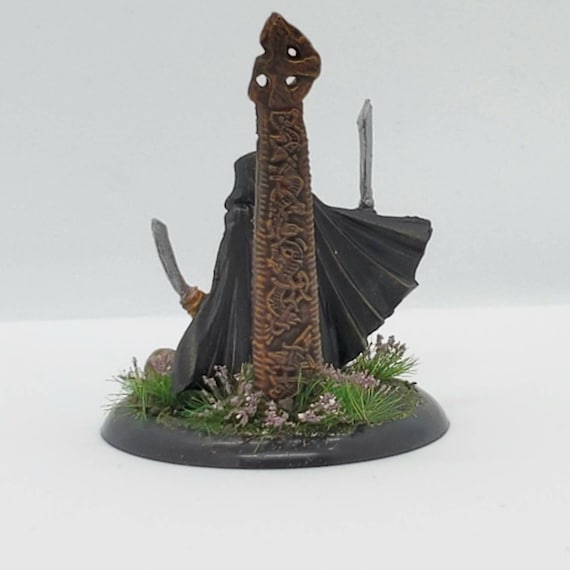This image features a detailed sculpture set on a wide, black base that resembles an upside-down bowl. At the base, grass and light purple foliage surround the sculpture, adding a touch of natural elements. The central focus of the sculpture is an ornate, light brown stone tower reaching approximately nine or ten feet in height, with intricate carvings and a broken Celtic cross at its apex. Standing behind this tower is a cloaked figure whose back is turned towards the viewer, draped in a black or dark green cape with a hood. The figure wields two swords, one in each hand—one with a brass-colored handle and the other with a black handle—which protrude from either side of the cape. The entire setup conveys a mystical or medieval aura, appearing as though it's a meticulously crafted toy or ceramic figure positioned on a gray platform for support.